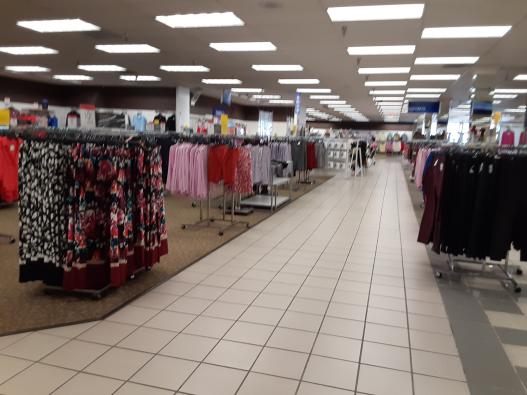In this detailed image of a well-lit store reminiscent of Target, we see a central aisle with white square tile flooring flanked by designated walking areas with distinct flooring patterns. The left walkway is carpeted and separated from the tile by a trim, while the right walkway features a gray thick stripe leading into a checkered gray and white carpet. Surrounding the central aisle are numerous racks predominantly displaying women's clothing. The racks on the left showcase an array of dresses and clothing items in colors such as purple, black, pink, red, garnet, and white. To the right, we see more racks with black clothing accented by a prominent purple shirt in the forefront. The store is brightly illuminated with a gray-tiled ceiling featuring regularly spaced square beams of artificial light. Although there are signs dispersed throughout the store, their details are out of focus. The overall scene lacks any visible shoppers, adding to a sense of tranquility within this bustling retail space.